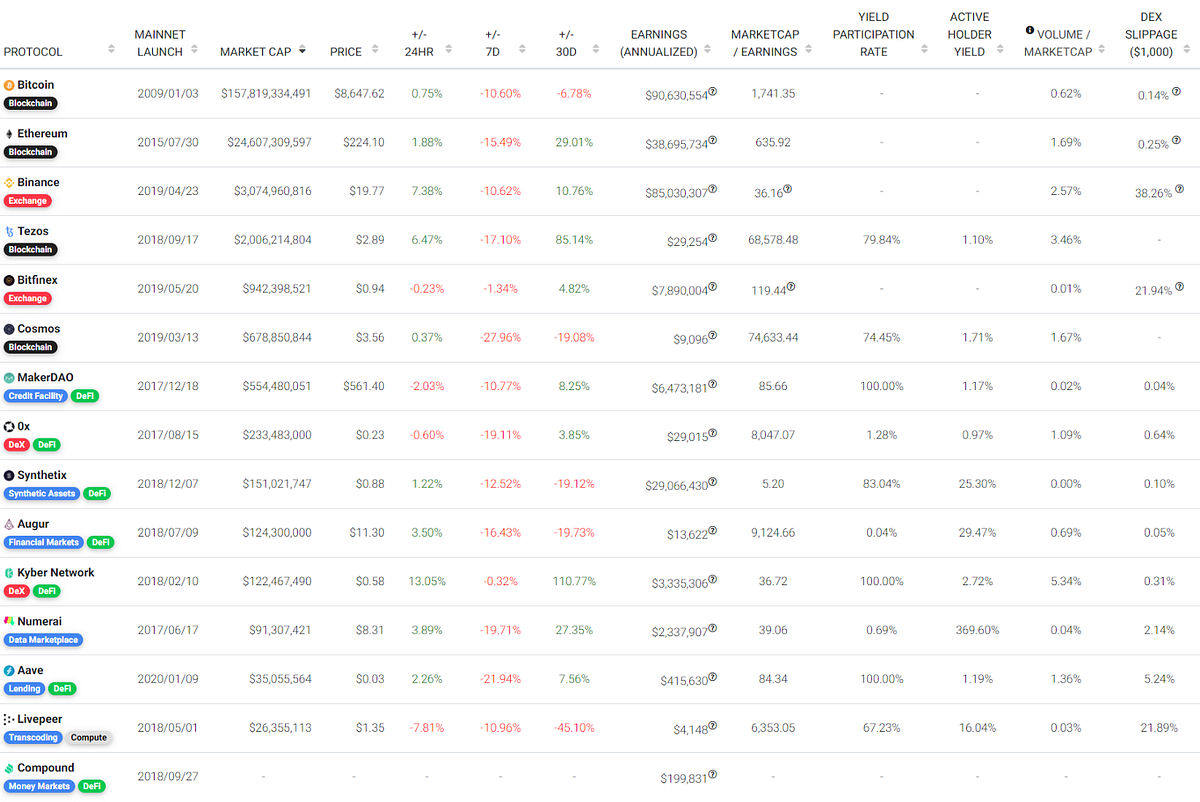The screenshot captures a comprehensive financial dashboard from a website, presenting an extensive array of metrics in a vertically aligned structure. 

At the very top, a horizontal list begins with "Protocol," followed by "Main Net Launch," beneath which are multiple dates. Adjacent columns include "Market Cap" with corresponding dollar amounts for each entry and "Price," also listed in dollar values.

Next, a column labeled "24 Hour" displays percentages indicating daily fluctuations, marked with plus or minus signs, displayed in green for gains and red for losses. This is succeeded by "± 7D," where all values, represented as red percentages, denote negative weekly performance. Following this, "± 30D" shows mixed green and red percentages indicating monthly performance, with some negative and some positive figures.

"Earnings (Annualized)" lists dollar amounts under each entry, while "Market Cap Earnings" presents simple numerical data. "Yield Participation Rate" features sporadic entries, either blank or represented as percentages, next to "Active Holder Yield," which consistently lists percentages.

Further columns include "Volume Market Cap," detailed as percentage figures, and "DEX Slippage," which also features percentages, encapsulating the varied financial metrics in a detailed, structured, and color-coded manner.